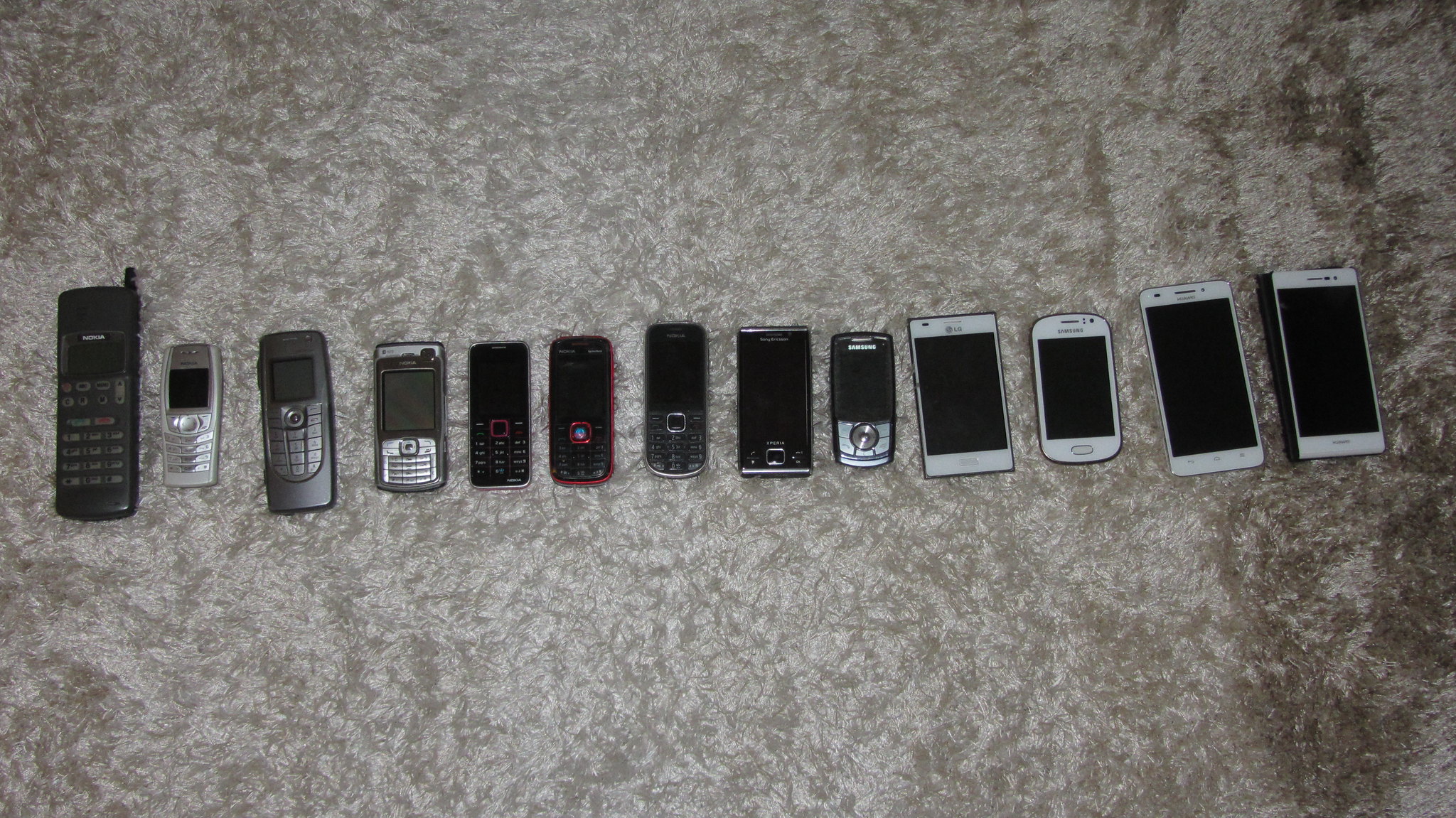This photo depicts a chronological lineup of 13 cell phones, likely representing the evolution of someone's personal collection over the past 20 or so years. The phones are laid out in a row on a gray carpet, starting from the left with an old, chunky model featuring a black keypad and antenna. As you move to the right, the phones become progressively smaller and more advanced. 

The sequence includes iconic Nokia brick phones, early PalmPilot models, and various flips phones. The color palette mainly consists of black, silver, and gray, with occasional red accents. The middle section features several silver and black bar phones, some with noticeable buttons and small screens. 

Towards the right end, the phones transition into modern smartphones with flat touchscreens, including what appear to be Android devices or iPhones, characterized by black screens surrounded by white borders. The final two phones are the largest and most recent, underscoring the leap in technology and design aesthetics over the years. The detailed arrangement on the carpeted floor provides a fascinating snapshot of the rapid evolution of mobile technology.